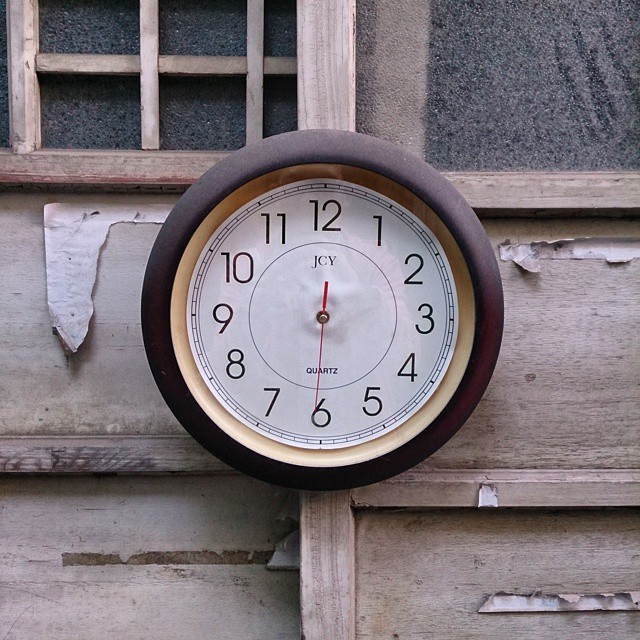This photograph captures a close-up view of a vintage clock hanging on a weathered wooden wall that appears to be the exterior of an old building. The clock features a dark brown, possibly metal or worn-out plastic exterior rim, along with a gold interior trim that frames its white face. The face of the clock displays black numbers 1 through 12 arranged in a circular pattern, with the brand name "JCY" and the word "quartz" prominently displayed in black near the center. Notably, the clock is missing its hour and minute hands, leaving only a slender red second hand, which is positioned at the 31-second mark. The white face looks slightly warped, suggesting that it might have been exposed to moisture at some point. The wooden wall behind the clock shows signs of age, with peeling paper and light-colored, worn wood, adding to the rustic charm of the scene. In the background, part of a frosted glass window is visible, further indicating the deteriorating state of this old structure.